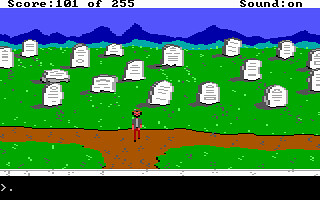In the top left corner, the screen displays the score: "101255". The top right corner shows "Sound: ON". A white bar runs across the bottom, resembling a command line with a chevron at the end. Above the command line, there's a thin white line at the top of it. The scene appears to be set in a cemetery, with a man walking along a crossroads. The road stretches horizontally from left to right, with another segment extending towards the bottom of the image. The ground is predominantly covered in grass. Two gravestones are visible, both white with inscriptions on them. The sky transitions from light blue to dark blue with patches of lighter blue scattered throughout. The entire image has a pixelated, video game aesthetic.